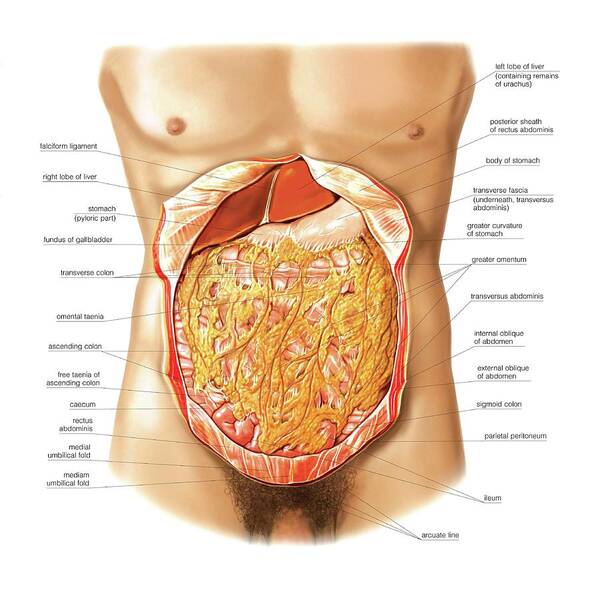This intricate medical illustration depicts the torso of a naked, white male from just below the chest, including the nipples, down to the top of the penis and partially the testicles. The skin of the torso is meticulously torn away and folded open, revealing the complex anatomy beneath. The drawing mainly focuses on the abdominal region, showcasing detailed inner structures such as the stomach, intestines, liver, and various muscles like the transversal abdominus and the internal oblique of the abdomen. Various parts are labeled with small, somewhat difficult-to-read black font in Latin, and arrows point to each corresponding anatomical feature. The background of the image is white, emphasizing that it is a precisely rendered drawing rather than a photograph, with a watercolor-like quality. Notably, the male figure also displays brown nipples and pubic hair, enhancing the realism of the illustration.